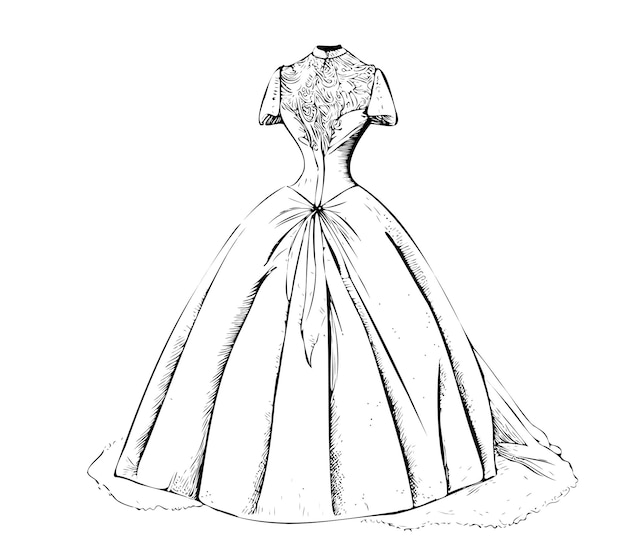This black-and-white sketch depicts a historically-styled gown displayed upright without a visible wearer or display stand. The dress features a tightly cinched, incredibly tiny waist, accentuating the intricate and ornate bodice that extends from the chest to the middle of the ribs. The bodice boasts an elaborate lace-like pattern, adding to its historical charm. The gown flares out dramatically, forming a bell-shaped hoop-style skirt that extends as wide as a person's outstretched arms. At the top, the dress comes up to a collar at the neck and has short, puffy sleeves that hang down, suggesting they would be larger when filled by arms. The sleeves exhibit a bell-shaped puffiness, contributing to the dress's voluminous appearance. Below the waist, the fabric gathers in a ruching style, potentially adorned by a central button, and a piece of fabric in the front appears to cinch off the main dress. Additionally, a train flows out and swirls around the bottom, adding elegance to the full-length gown, all set against a stark white background.